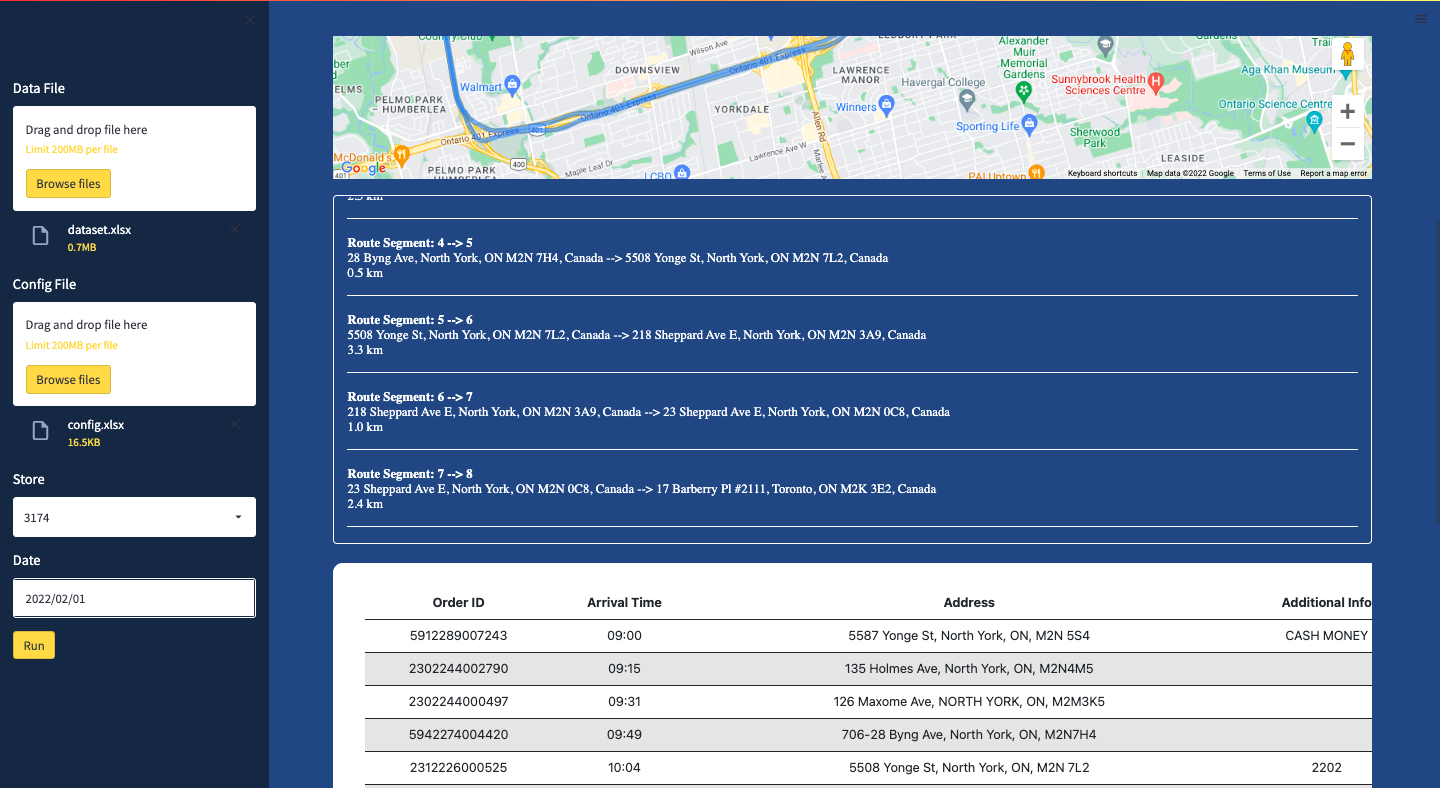In the image, there is a web page or application interface with a primary color scheme consisting of various shades of navy blue. The top half of the page features a map, highlighting regions such as Downsview, Yorkdale, Lawrence Manor, Haverhill College, Boarding Life, and Sherwood Park. Below the map, there are lines indicating different addresses and route segments associated with these locations.

On the left side of the page, there is a dark navy blue pane labeled "Data File," which prompts users to drag and drop files up to a 200 MB limit. This pane includes a yellow "Browse Files" button for file selection. Additionally, there is a "Config File" section allowing for similar file interactions, as well as options labeled "Store," "Date," and a "Run" button.

Below the map, the page displays detailed information including order IDs, addresses, and arrival times. This suggests that the interface is related to delivery or package management. For example, one of the entries lists Order ID 591-228-900-7243 with an arrival time of either 9 minutes or 9 o'clock (without specifying AM or PM), along with an address and additional information marked as "cash money." This entry implies the application is tracking deliveries or shipments, detailing order specifics and logistics.